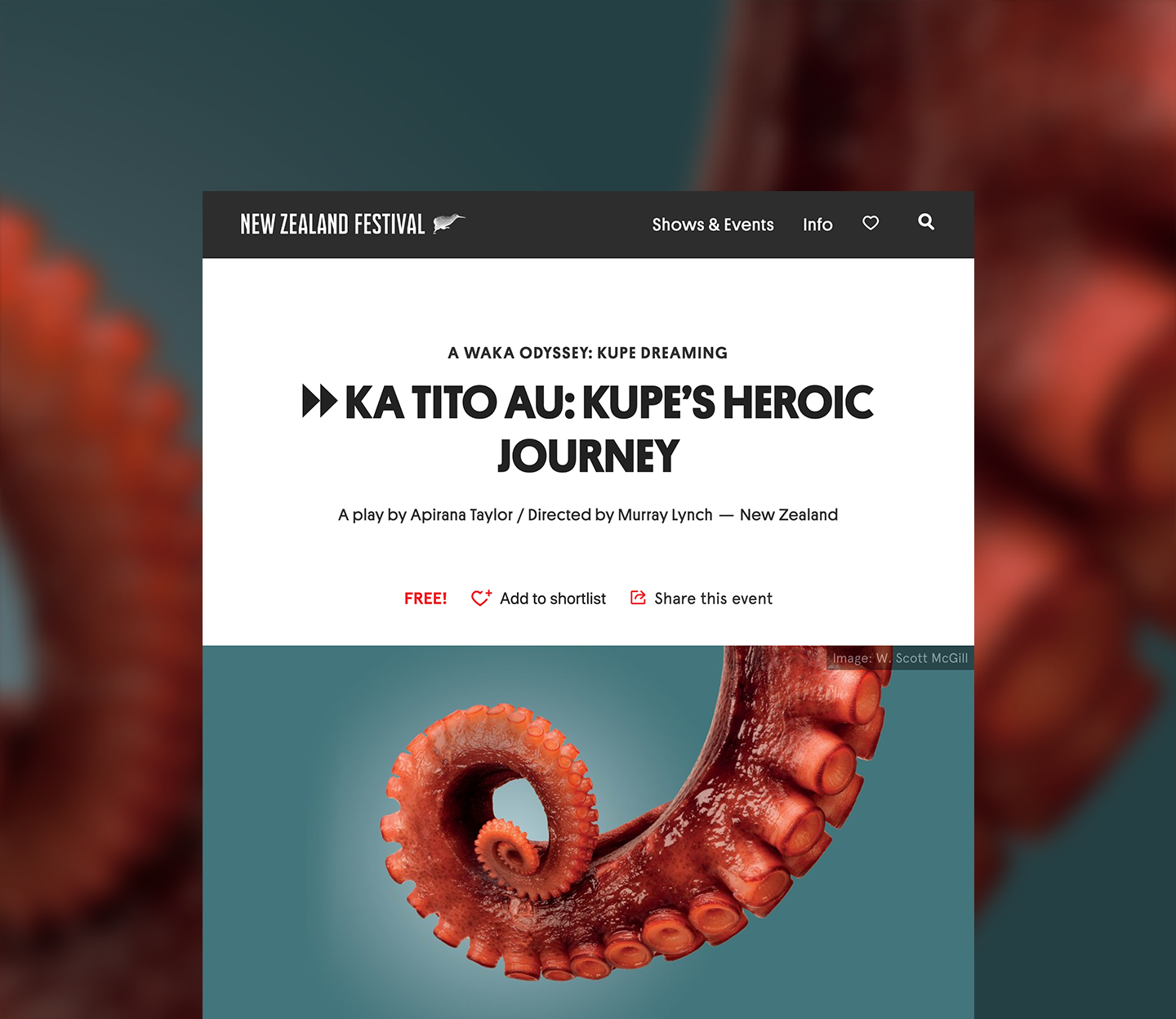A visually distinctive poster for the New Zealand Festival is presented, thoughtfully layered with multiple elements against a vibrant blue backdrop. The background features a deeply blurred image of an octopus tentacle, its details obscured to maintain focus on the foreground elements. 

Superimposed on this backdrop is a sleek grey panel. On the left side of this panel, the text boldly reads "New Zealand Festival." To the right, a list of icons provides quick access to "Shows and Events," "Info," a heart symbol for favorites, and a search icon. Just below this panel, a crisp white rectangle draws attention, prominently announcing "Waka Odyssey," a play by Asperano Taylor, directed by Murray Lynch. It clearly states that the event is free, with options to "Add to shortlist" or "Share this event."

Embedded below the white rectangle is a subsequent, more focused image showing the same blue background with a close-up of the octopus's tentacle, now clearly in focus. This sharp, detailed section reveals the intricacies of the tentacle, providing context to the previously blurry background and adding a visually engaging layer to the overall design.